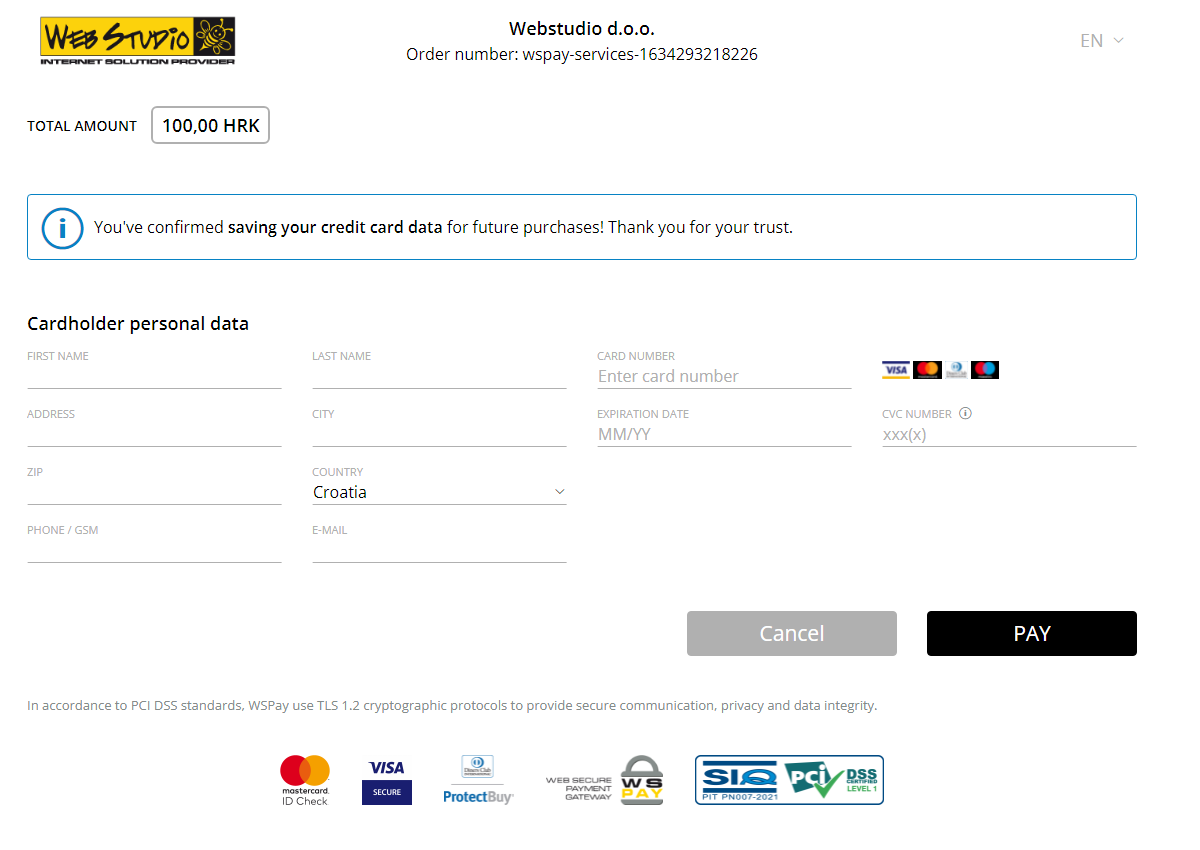Order Confirmation Overview for Web Studio Services

---

**Order Number:** 1634293218226EN  
**Total Amount:** 100 HRNC

You have successfully placed an order for web studio services. Your credit card details have been securely saved for future purchases, demonstrating your trust in our system.

**Cardholder Information:**

- **First Name:** [First Name]
- **Last Name:** [Last Name]
- **Address:** [Full Address]
- **City:** [City]
- **ZIP Code:** [ZIP]
- **Country:** Croatia
- **Phone:** [Phone Number]
- **Email:** [Email Address]

**Credit Card Information:**

- **Card Number:** [Card Number]
- **Expiration Date:** MM/YY
- **CVC:** XXX (protected)
- **Card Type:** Visa, MasterCard, or American Express

For your security, all transactions comply with PCI DSS standards. Communication is protected using Tillis 1.2 cryptographic protocols to ensure privacy and data integrity. Payment processing is safeguarded by WBSIQ PCI DSS certification.

Thank you for your trust and for choosing our services. If you need to cancel or require further assistance, please contact us.

**Payment Options:**

- Visa
- MasterCard
- American Express